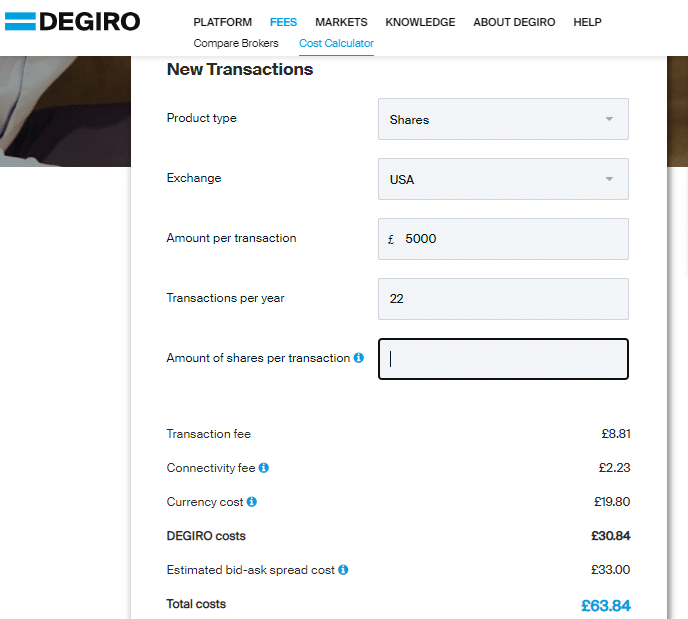The image shows a webpage from "The Giro," prominently displayed with the name "The Giro" in black text on the top left of the header, alongside a blue equal sign, symbolizing the brand. The header features several navigation tabs: "Platform Fees," "Market," "Knowledge About The Giro," and "Help." The background of the page is white, and the "Fees" tab is currently highlighted in blue, indicating it is selected, while the other tabs remain in black.

Under the "Fees" section, there are options to "Compare Brokers" and a "Cost Calculator," with the latter currently chosen, hence displayed in blue. The "Cost Calculator" encompasses various fields: "New Transaction," "Product Type," "Shares," with a dropdown menu for selecting the product type. The "Exchange" field is set to "USA," the "Amount per Transaction" is 5,000 euros, "Transactions per Year" is 22, and the "Amount of Shares per Transaction" field is left empty.

Toward the bottom of the page, the following costs are detailed:
- Transaction Fee: 8.81 euros
- Connectivity Fee: 2.23 euros
- Currency Cost: 19.80 euros
- The Giro Cost: 3.84 euros
- Estimated Bid-Ask Spread Cost: 33.00 euros
- Total Cost: 63.84 euros

The total cost is prominently positioned on the bottom right, highlighted in blue.